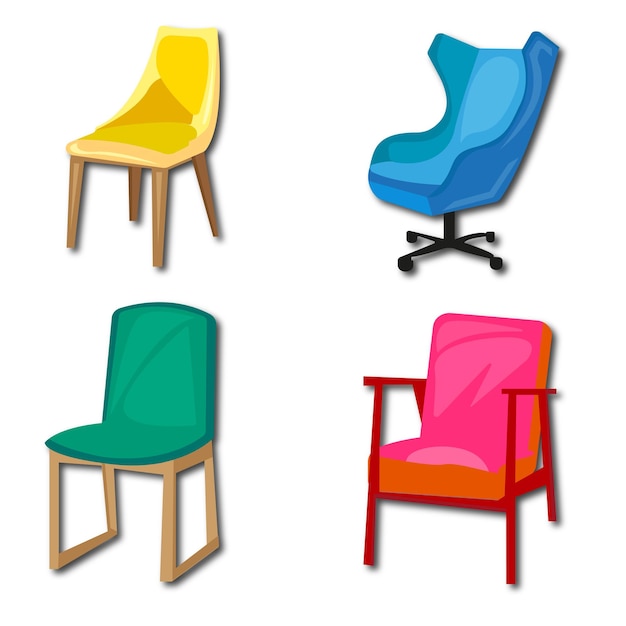This is a detailed illustration of four chairs against a white background, each depicted in a unique style and color. The top left chair, which resembles school furniture, features a yellow plastic seat and four brown wooden legs. The top right chair is a blue lounge chair with a neck rest and a black rolling wheel base, oriented towards the left. Positioned on the bottom left is a turquoise chair with two beige wooden legs. Finally, the bottom right showcases an armchair with a hot pink seat, distinct orange cushioning, and four red legs. All chairs appear to be digitally drawn, possibly AI-generated, with no additional objects, text, or living beings included, and each chair is slightly facing to the left.